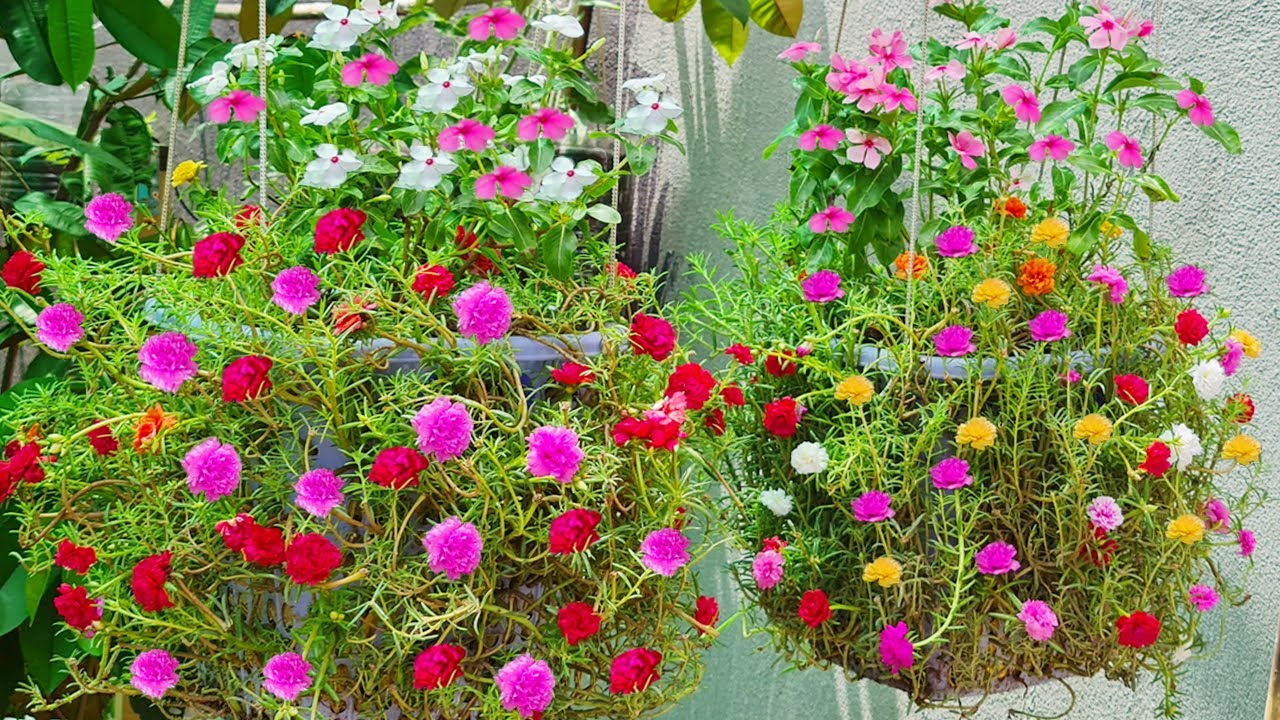This is a vibrant color photograph of two hanging flower baskets set against a white stucco wall. The baskets, suspended by white strings, are richly adorned with a variety of blooming flowers that seem to be growing through and around them, almost concealing the baskets entirely. In the left basket, bright pink and red carnations dominate, interspersed with white and pink-petaled flowers with green leaves at the top, adding an extra layer of lushness. Beneath these, trailing branches showcase more pink and purple puffy blossoms. Similarly, the right basket is a colorful mix, featuring yellow, white, and pink carnations coupled with light and dark pink petaled flowers, creating a harmonious blend of hues. The meticulous care given to these plants is evident in their full, vibrant blooms. The scene suggests a warm climate, perfect for nurturing such a diverse array of flowers, making it a captivating focal point that draws the viewer’s eye immediately.